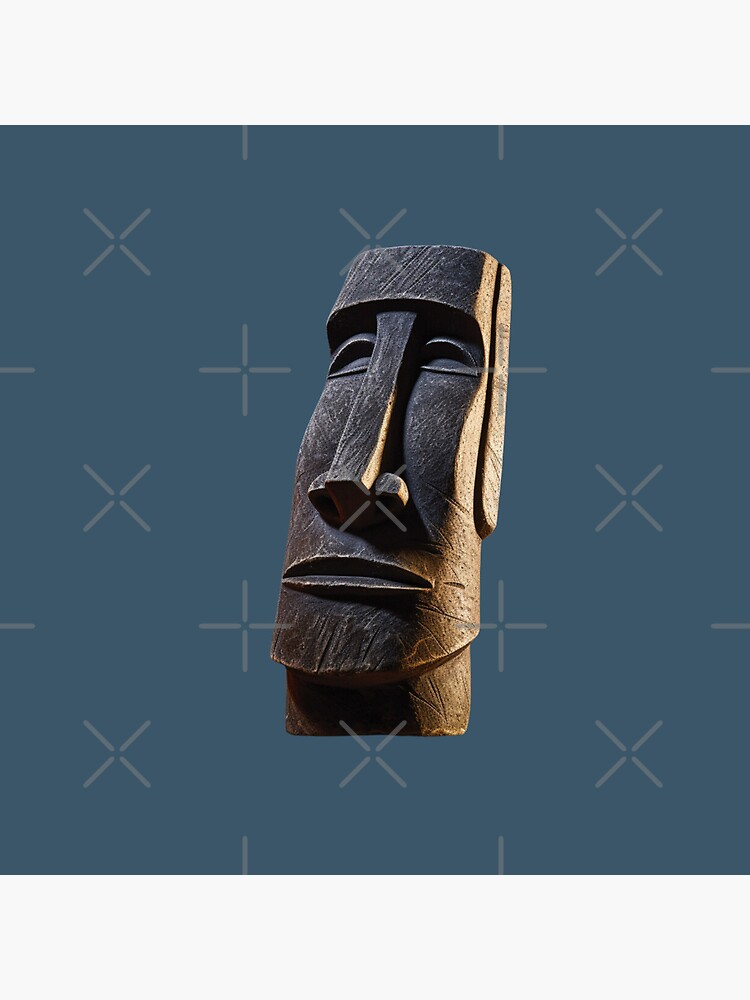The image showcases a large, intricately carved statue resembling the iconic Easter Island heads, yet appearing notably new and unworn, suggesting it is an artwork displayed indoors, potentially in a museum setting. The statue is characterized by a long, flat nose, slit-like eyes and mouth, and additional facial details including nostrils and lips, all sculpted into a brown material that appears to be either wood or stone. It features design elements that vaguely resemble a helmet with flaps akin to ears extending down the sides. The background of the image is a teal blue color, adorned with rows of alternating X's and pluses, creating a patterned backdrop that frames the statue centrally in what could be described as a neatly spaced, artistic manner. The X's are depicted as not fully connected in the center, adding a subtle complexity to the design that enhances the overall composition of the image.